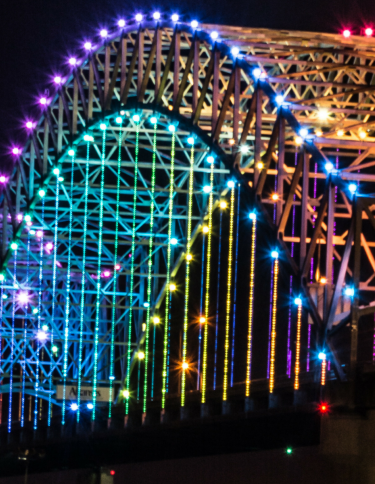The image captures a large, rounded structure at night, which initially resembles a roller coaster but is more likely to be a bridge due to its wide arching foundation. The structure is prominently lit with vibrant, multicolored lights that range from bright purple around the archway to a gradient of turquoise, blue, green, yellow, and orange extending downwards. These lights festively decorate the bridge, making it an eye-catching feature against a very dark, almost black background. There's also a sign in the bottom left of the image, although it's not readable. The overall scene suggests a decorative display, possibly set up to enhance the attractiveness of the bridge or for a special occasion.